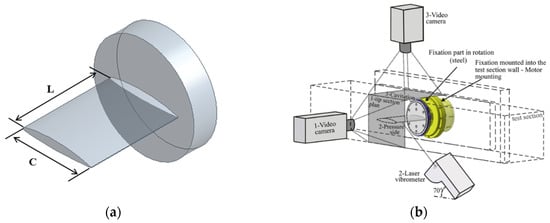The image features a white background with two detailed diagrams side-by-side. On the left, a gray, almost upright cylinder slightly leaning back has an L labeled on its left side and a C on its bottom side. A flat, gray rectangle stands behind it. On the right, a more complex structure is depicted. This consists of a vertical rectangle connected to a horizontal flat rectangle at the top, which is in turn connected to another vertical rectangle on one end. Beneath this assembly, there is a yellow cylinder, and the entire setup is shaded in gray. This structure is labeled as a video camera system, with annotations mentioning components like a fixation part in rotation, a steel fixation mounted into a test section wall, motor mounting, and a three-layer vibrometer. This second diagram suggests a sophisticated camera arrangement for capturing different angles, possibly indicating a specialized video system setup.